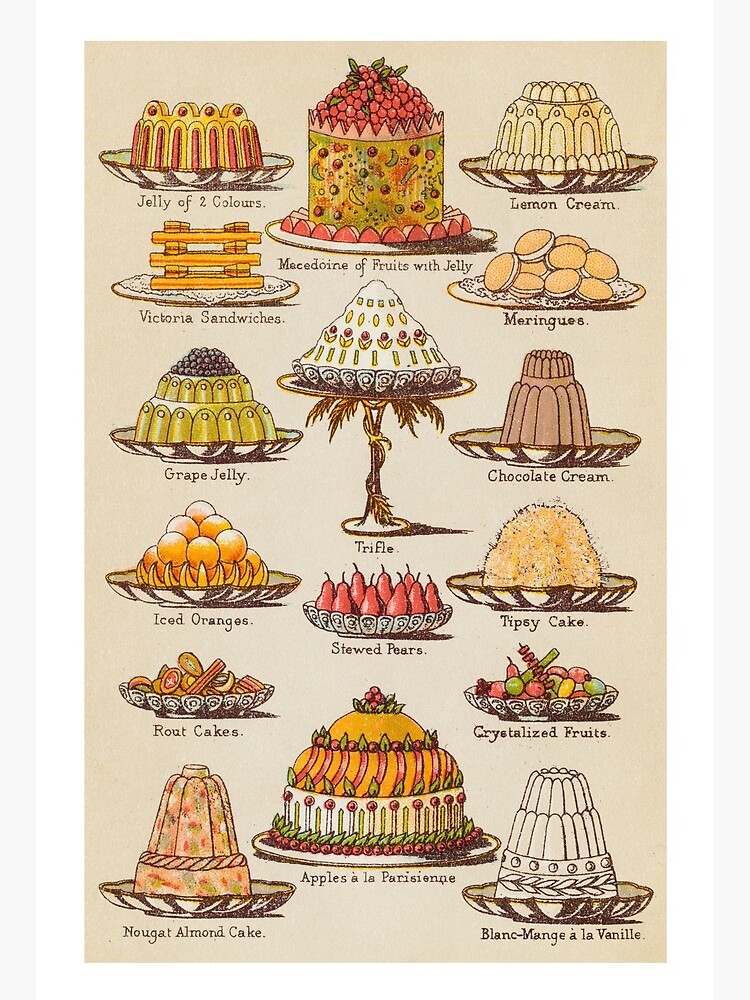This is a detailed illustration showcasing an array of colorful cakes and desserts, all labeled at the bottom in black text for easy identification. The variety includes jelly of two colors, Victoria sandwiches, grape jelly, iced oranges, raut cakes, nougat almond cake, macedoine of fruits with jelly, trifle, stewed pears, apples à la Parisienne, lemon cream, meringue, chocolate cream, tipsy cake, crystallized fruit, and blancmange à la vanille. The desserts are artfully arranged on plates against a light beige background. Notably, the Victoria sandwiches are depicted as three-layered treats, adding to the visual appeal. This beautifully detailed image evokes a sense of indulgence and culinary delight, making the viewer almost taste the scrumptious array, even through the canvas. The light brown tannish backdrop complements the vividly colored desserts, enhancing their visual appeal. The illustration might be a snippet from a web page, though the web address is not provided.